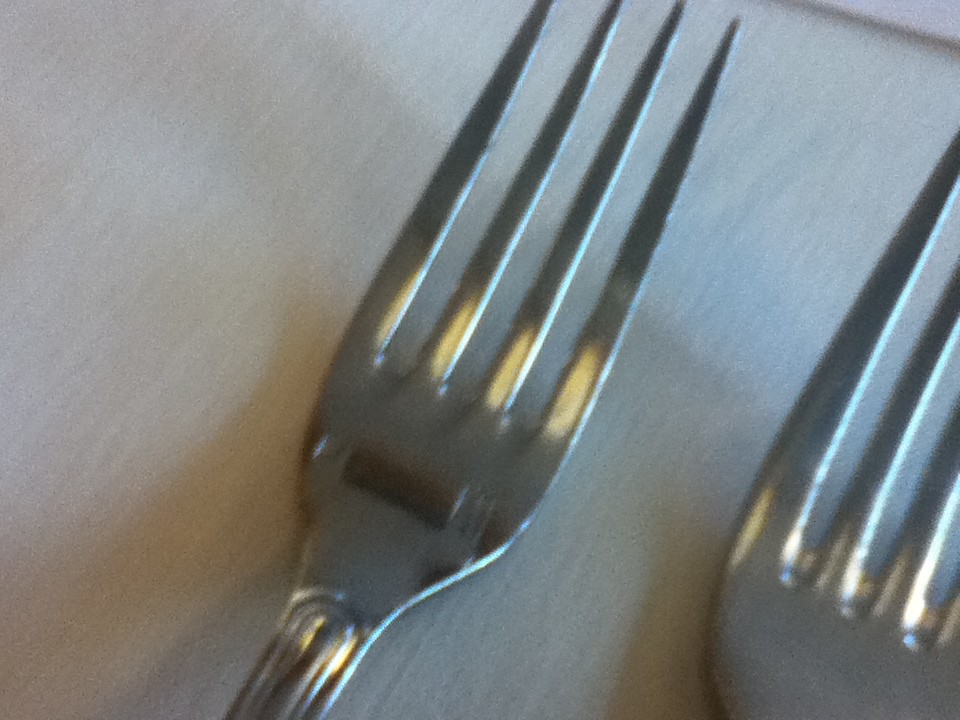The image depicts a close-up, moderately out-of-focus shot of two silver stainless steel forks on an off-white tablecloth or possibly a light-colored surface with subtle wood grain. The photo, wider than it is tall, captures predominantly the heads and tines of the forks, with both forks oriented in the one o'clock direction. The left fork, occupying a position roughly a third from the left edge, shows its four tines clearly and features a coppery, horizontal rectangle near the base of the prongs, indicating a reflection or glare from the light source. The right fork is only partially visible, showing just a few of its tines in the lower right-hand corner. Light from behind the camera casts a shadow across the surface, creating reflections on the forks and adding to the overall soft, slightly blurred aesthetic of the photograph.